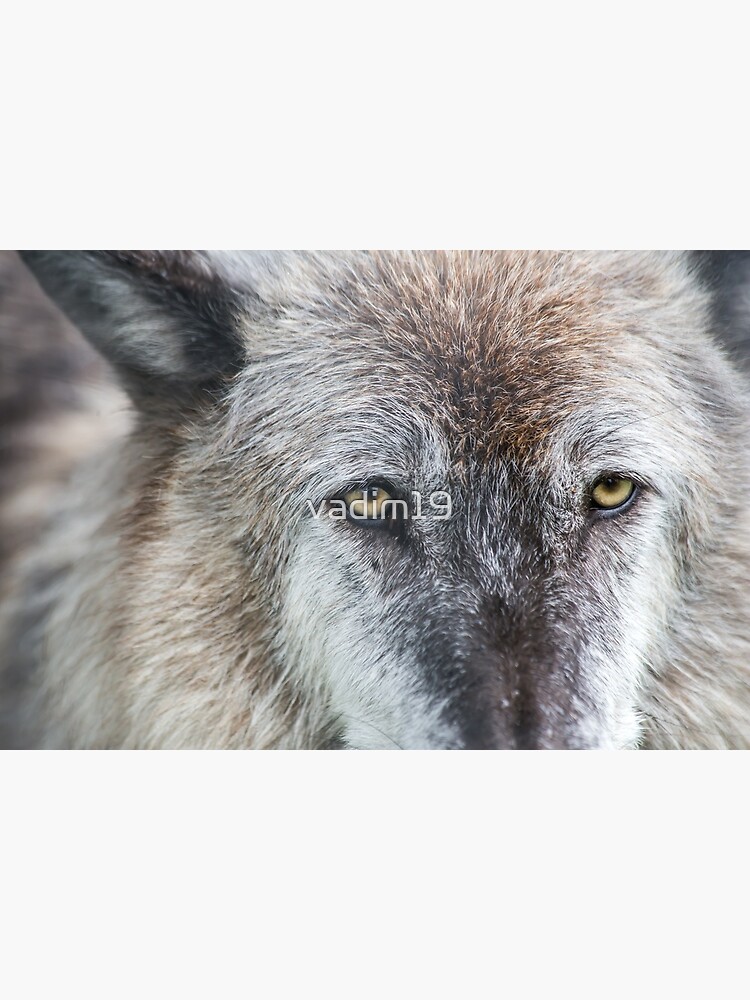The image is a striking close-up of the eyes of a wolf, though it's cropped so tightly that the full face isn't visible, with the nose and top of the ears out of the frame. The wolf's half-lidded, amber-colored eyes gaze slightly off to the distance, giving the impression that it might be just waking up, falling asleep, or possibly unwell. The fur, which is high quality and lush, features a mix of red, brown, tan, gray, and black tones, suggesting a cold setting, possibly with some snowflakes visible on the nose. The single visible ear is sharp, although the other is cut off from view. Overlaid on the wolf's left eye is a watermark text reading "V-A-D-I-M 19," identifying the photographer. The background is blurry, further emphasizing the detailed and intimate focus on the wolf's beautiful, enigmatic eyes.